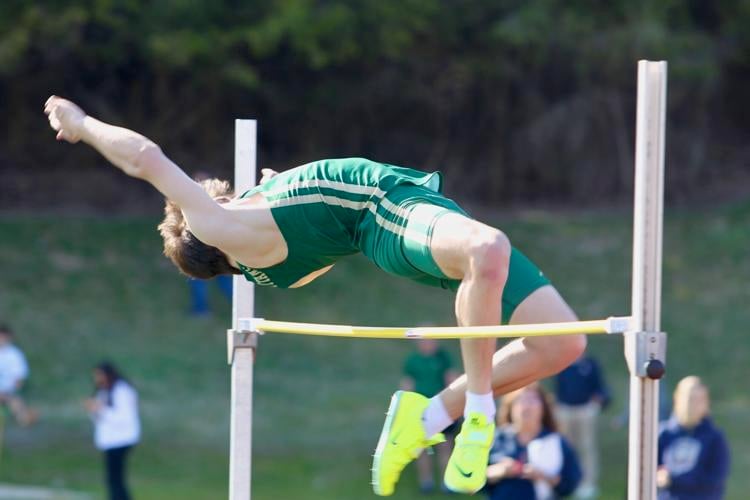The image captures a dynamic moment of a young, well-muscled white male athlete mid-air as he executes a high jump on an outdoor athletic field. Dressed in a vibrant green track outfit with distinctive white stripes running from his tank top down to his shorts, the athlete sports neon yellow sneakers and white socks. His back arches gracefully over a plastic yellow high jump bar held up by two metal vertical beams, showcasing his exceptional athletic form. The scene is enriched by the blurred background, featuring a green grassy hill leading up to a dense tree line, and sparse spectators observing from a small hill. Overall, it's an action-packed photograph highlighting the skill and poise required for the high jump.